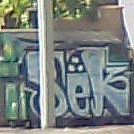The image appears to showcase an outdoor scene during daylight, capturing every detail clearly. Central to the composition is a white pillar extending vertically. In the background, there's an old, possibly brick wall that includes spray-painted graffiti reading "S.E.K" with a capital "S" followed by lowercase "e" and "k". This graffiti is predominantly blue and white in color. The top left corner to the middle of the image features some plants. Despite the image being small, these elements are distinctly visible.